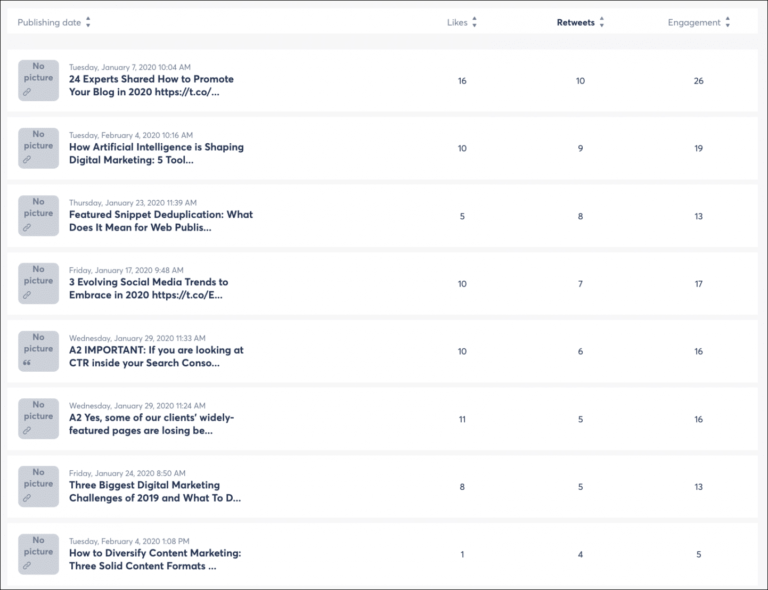The image depicts a rectangular, white-background interface with several columns labeled Publish Date, Likes, Retweets, and Engagement. The first column, Publish Date, is grayed out and features an up and down button with the text “Publish Date.” Adjacent to it, the Likes column is also grayed out, while the Retweets column is highlighted in dark black, indicating that it is currently active or selected. The far-right column, Engagement, is grayed out and also includes an up and down button labeled “Engagement.”

Each row under these headers corresponds to a different article, with no accompanying images, only gray boxes marked “No Picture.” The content appears to be a list of social media or blog posts. The first row highlights an article titled "24 Experts Share How to Promote Your Blog in 2020," along with a partial URL and a date. Under the Likes column, it registers 16 likes; the Retweets column shows 10 retweets; and the Engagement column lists 26 engagements.

Subsequent rows follow the same format, such as an article titled "How Artificial Intelligence is Shaping Digital Marketing," published on Tuesday, February 4, 2020, with 10 likes and partial title visibility. Altogether, there are around 8 to 9 listed articles, each with corresponding engagement metrics under the four mentioned columns.